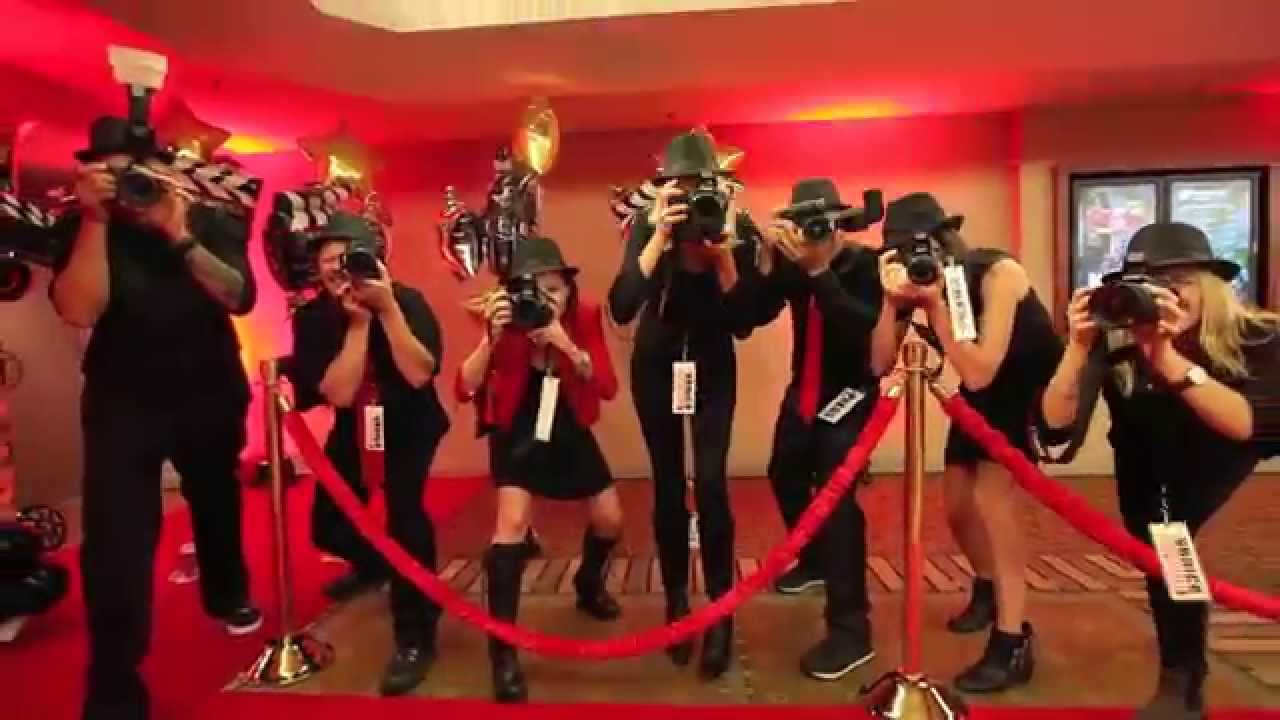This photograph captures the perspective of a celebrity facing a swarm of paparazzi. Half a dozen photographers, men and women alike, stand on the other side of a red velvet rope secured between two gold posts, with their cameras focused intently, obstructing their faces and poised in various crouched positions. Dressed predominantly in black, one of the women sports a red top, while a man is distinguished by his red tie. The background consists of a red wall adorned with occasional black and white elements, and the upper ceiling is bathed in pinkish-orange lighting. The floor is wooden, adding a touch of brown to the scene. Each photographer wears a name tag indicating "Press," emphasizing the staged, almost surreal nature of this setup, reminiscent of a celebrity event.